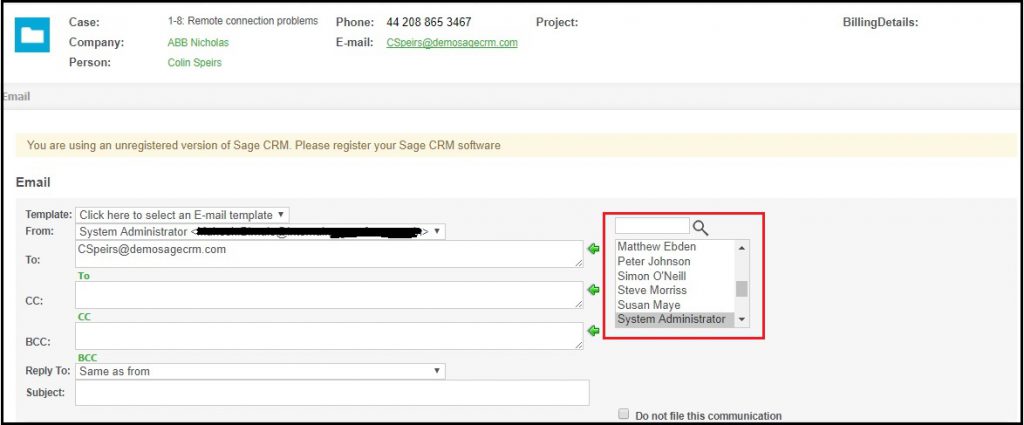Screenshot of a Customer Problem Tracking System Interface

The screenshot depicts a Customer Problem Tracking System, possibly within Sage CRM software, focusing on a case labeled "1-8 Remote Connection Problems" for company "ABB Nicholas." The interface is as follows:

1. **Icon and Header:**
   - **Upper Left Corner:** A turquoise square icon with a white file folder image.
   - **Header:** Displaying "Case 1-8 Remote Connection Problems."

2. **Customer Details:**
   - **Company:** ABB Nicholas
   - **Person:** Colin Spears
   - **Contact Information:**
     - **Phone Number:** (provided but obscured in the image)
     - **Email:** (email address provided but not displayed for privacy)

3. **Project and Billing Details:**
   - **Project:** No information provided.
   - **Billing Details:** No information provided.

4. **Email Section:**
   - **Email Section Header:** Marked by a gray bar labeled "Email."
   - **Software Notification:** "You are using an unregistered version of Sage CRM. Please register your Sage CRM software."
   - **Email Composition Area:**
     - **Template Selection:** "Template. Click here to select an email template from System Administrator." However, this section is scratched out and not fully visible.
     - **Recipient:** Addressed to C Spears, the email address is provided.
     - **CC/BCC Options:** A red box highlights a series of selectable names that can be transferred to the CC or BCC fields, though the reason for this highlight is unclear.

The overall layout is structured to manage customer issues efficiently, but certain areas like project details and billing are left unfilled. Additionally, the email template section is obscured, indicating restricted visibility.